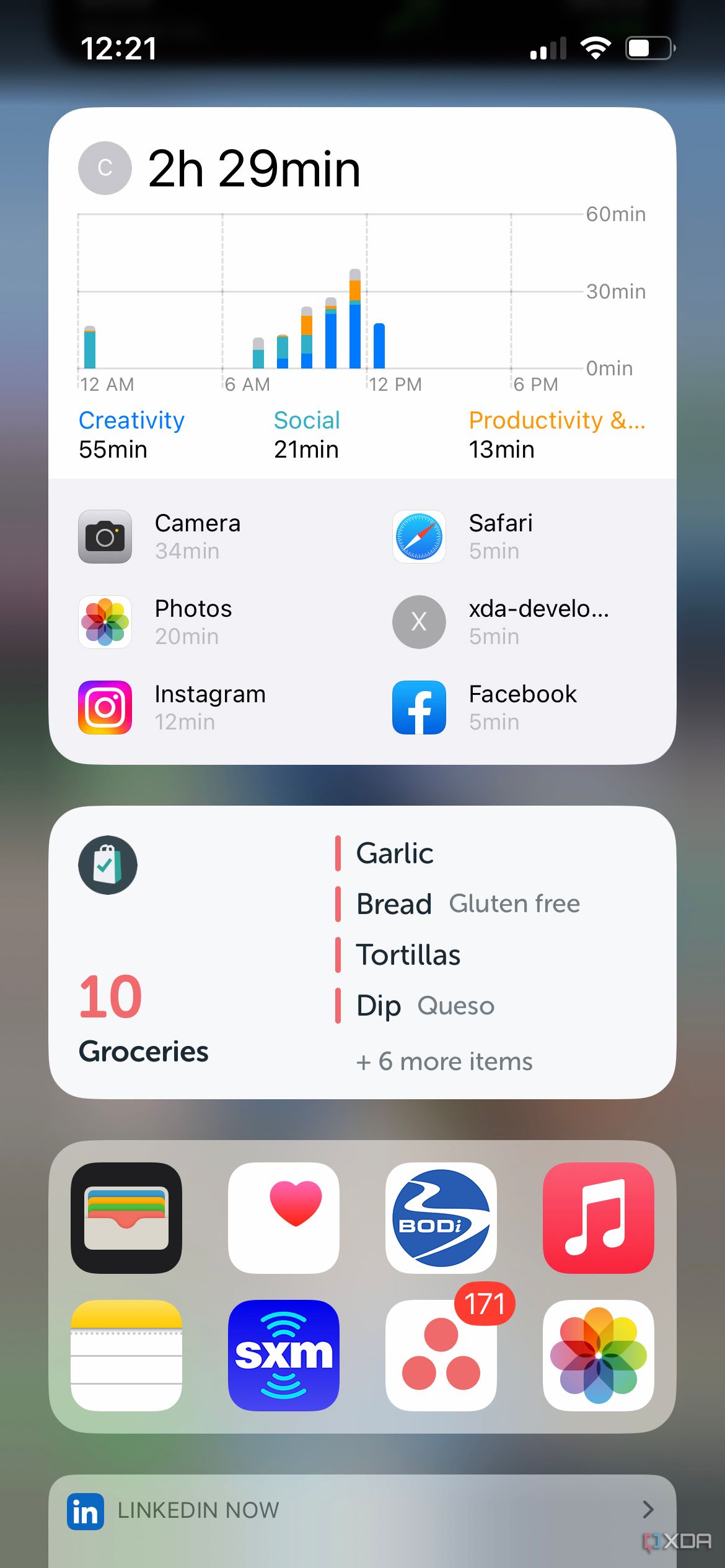Screenshot of a smartphone home screen displaying various widgets and icons. 

In the upper left corner, the time is shown as 12:21. In the upper right, icons for cell phone reception, Wi-Fi, and battery status are visible. Below these icons is a widget displaying app usage statistics. This widget shows a breakdown of the phone's use over a time span, with a graph indicating activity at intervals of 12 a.m., 6 a.m., 12 p.m., and 6 p.m. The graph shows that the total screen time is 2 hours and 29 minutes, broken down into categories: 55 minutes for creativity, 21 minutes for social, and 13 minutes for productivity. Additionally, it lists the most accessed apps: Camera, Photos, Instagram, Safari, XDA Developers, and Facebook.

The next section contains another widget, which appears to be a list-making app, likely a grocery list, although further details of the list content are not visible.